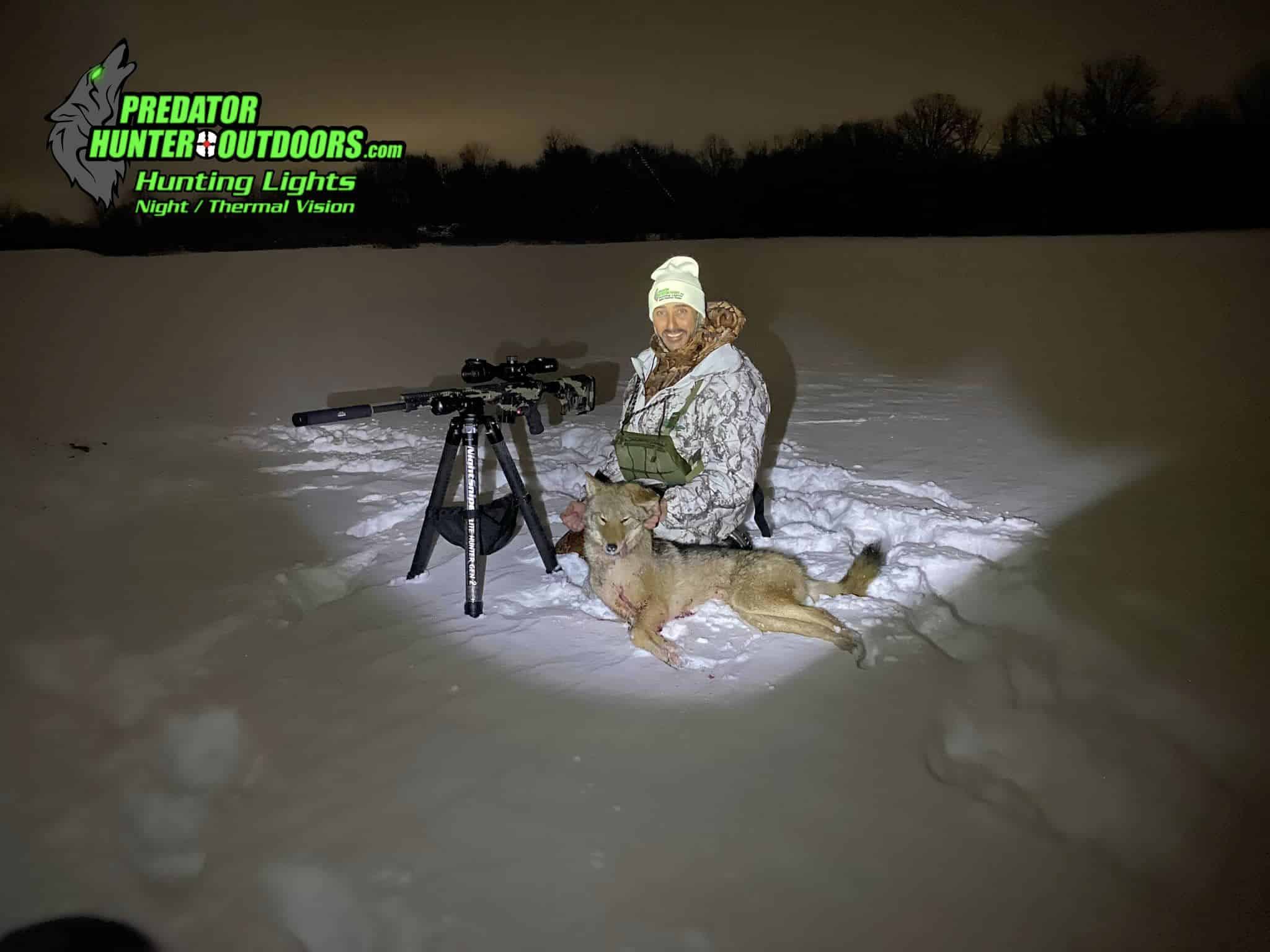In the dead of night, under a dark gray sky framed by a distant black tree line, a striking advertisement unfolds in a blanket of pristine white snow. The center of the image spotlights a hunter, outfitted in white camouflage with a white beanie, clearly displaying a mustache and possibly a beard. The man is kneeling beside a recently shot small wolf, lifting its head in a victorious pose. The scene is well illuminated, focusing on the man, the wolf, and his sophisticated hunting rifle mounted on a tripod equipped with a black silencer and large scope. Tracks in the snow hint at movement, leading up to this moment. The top left corner of the image features green text that promotes PredatorHunterOutdoors.com with the keywords: Hunting Lights, Night, and Thermal Vision.